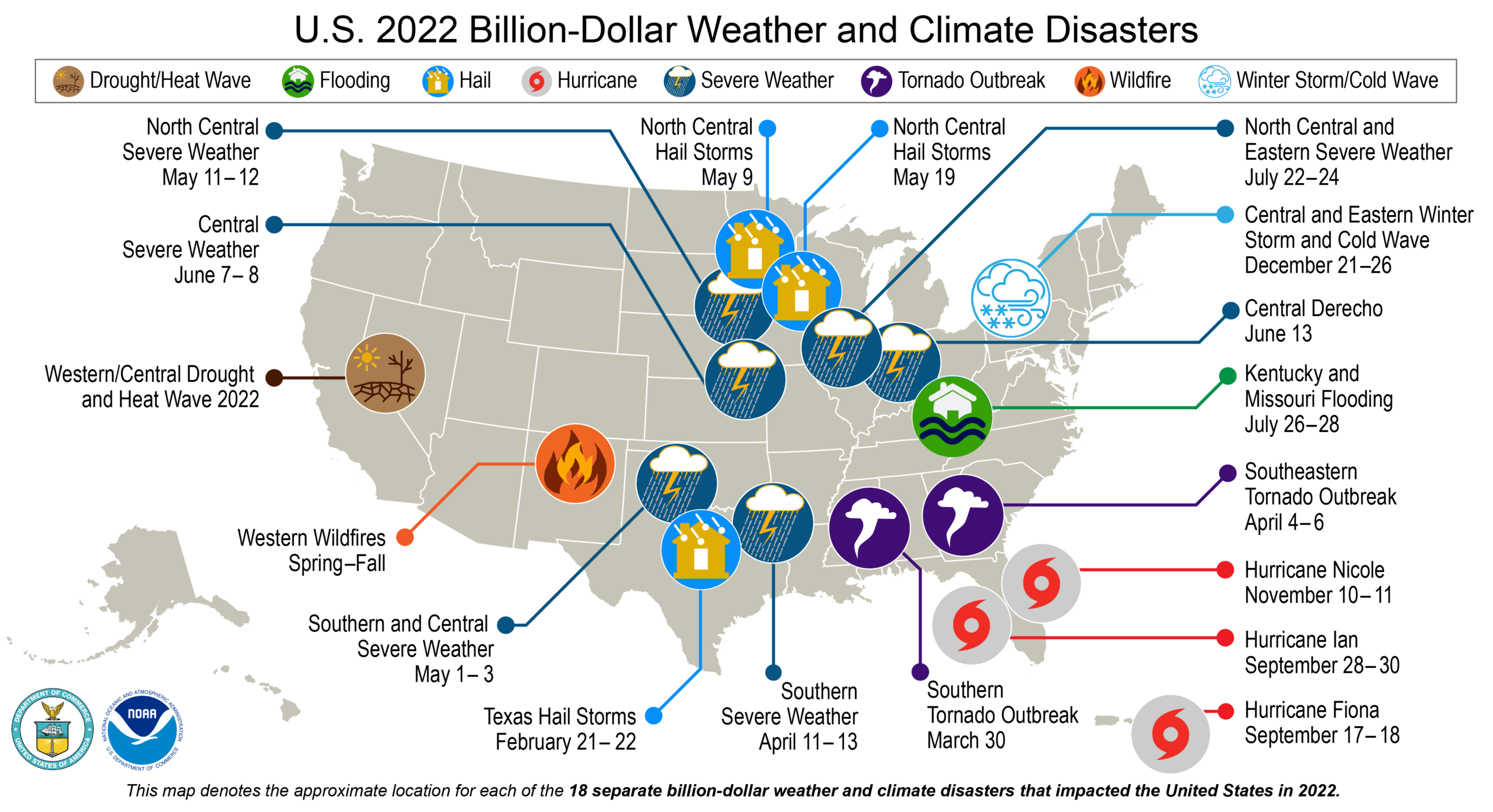The image depicts a detailed map of the United States titled "U.S. 2022 Billion-Dollar Weather and Climate Disasters." The map is grayed out and features a white background. Scattered across the map are various circular icons indicating the locations and types of significant weather and climate disasters that occurred in 2022, each costing over a billion dollars in damages. 

At the top of the map, a legend categorizes the disasters using different colored labels: brown for drought and heatwaves, green for flooding, blue and orange for hail, red for hurricanes, a rainbow-like color for severe storms, purple for tornado outbreaks, orange for wildfires, and light blue for winter storms and cold waves. 

Descriptions and dates of specific events are provided, such as: North Central Hail Storms on May 19th, Southeastern Tornado Outbreak from April 4th to 6th, and multiple hurricanes like Hurricane Nicole on November 10th-11th, Hurricane Ian on September 28th-30th, and Hurricane Fiona on September 17th-18th. Accompanying each icon are details like "North Central and Eastern Severe Weather, July 22nd-23rd," or "Central and Eastern Winter Storm and Cold Wave, December 21st-26th." 

The bottom of the map states, "This map denotes the approximate location for each of the 18 separate billion-dollar weather and climate disasters that impacted the United States in 2022."